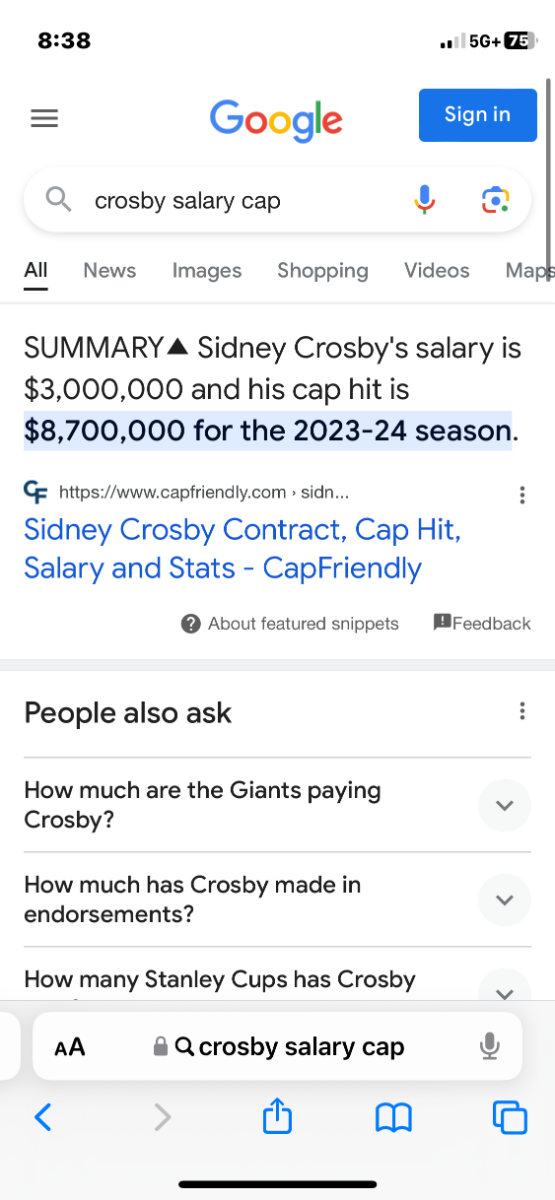The image depicts a screenshot taken on a smartphone of a Google search for "Crosby Salary Cap." The search results page shows the "All" section underlined in black, with additional tabs visible, including "News," "Images," "Shopping," "Videos," and "Maps." Prominently highlighted in blue is information stating that Sidney Crosby's salary for the 2023-24 season is $3,000,000, and his cap hit is $8,700,000. Below this highlighted section is a clickable link in blue font titled "Sidney Crosby contract cap hit salary and stats - CapFriendly." Further down, the "People also ask" section features questions such as "How much are the Giants paying Crosby?", "How much has Crosby made in endorsements?", and "How many Stanley Cups has Crosby?" The screen is partially cut off at the bottom, truncating additional information. In the middle of the image, there is a small snippet with a question mark icon and text about "Featured Snippets," along with a feedback option.